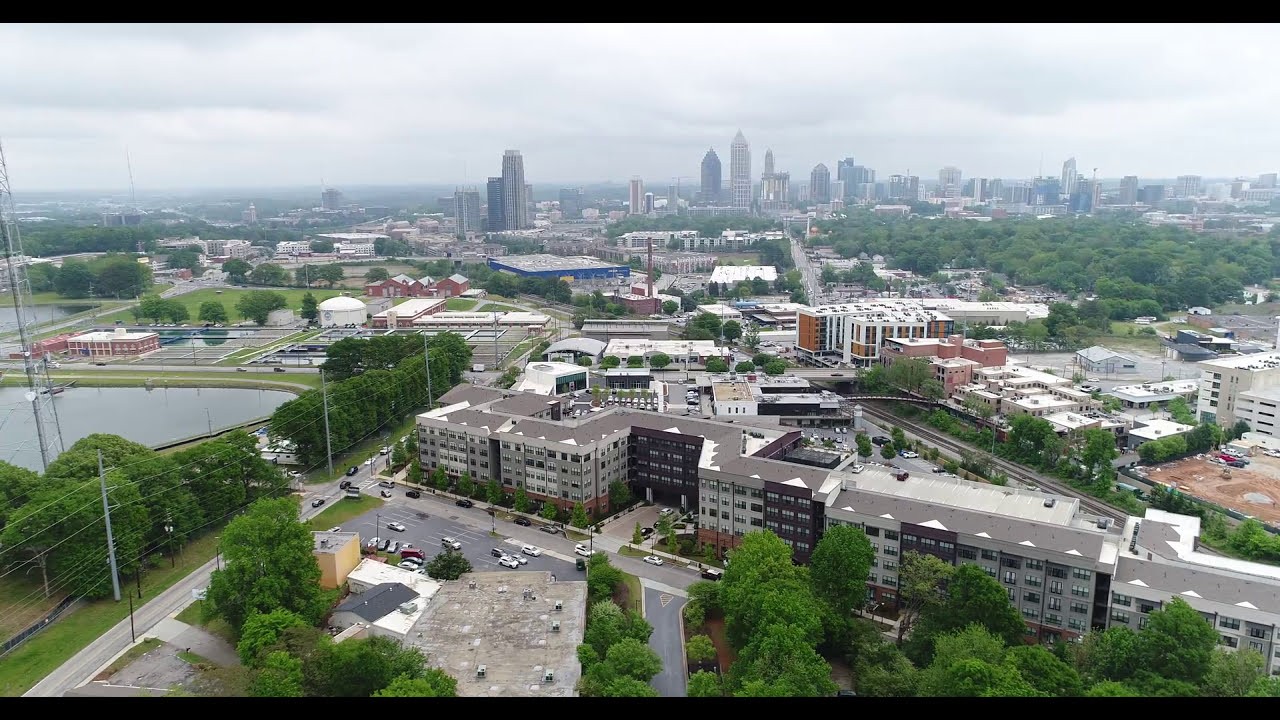This overhead aerial photograph, framed with black horizontal bars at the top and bottom, captures a detailed view of a suburban town just outside of a larger city. The town is characterized by rows of residential apartment buildings lined along a street that runs at a 60-degree angle from the middle-left to the lower-right of the image. Leading from the town, a perpendicular street is flanked by a dense row of green-leafed trees and shrubs, extending towards a body of water, likely a lake or pond, on the far left side of the image.

In the foreground, a parking area and the rooftops of more apartment buildings can be seen, immersed in a dense canopy of tall green trees. Behind these buildings, the residential area continues with more streets and buildings as the scene stretches towards the horizon. As the image progresses into the background, the suburban landscape gives way to a city skyline, populated by various architectural styles, including peaked and square-topped high-rise buildings. 

The tallest, densely packed skyscrapers are concentrated more towards the upper right of the image while the upper left shows sparse development. The background view hints at a hazy skyline with an indication of mountains and a hill in the far distance. The cityscape is interspersed with lampposts, electrical poles, mobile towers, and roads with cars, with numerous trees bordering these structures. Additionally, elements such as parks, an airport, and possibly a stadium or construction site form part of the distant landscape. The sky above is grayish-blue, dotted with puffy white clouds, creating a serene backdrop for this diverse and bustling urban area.